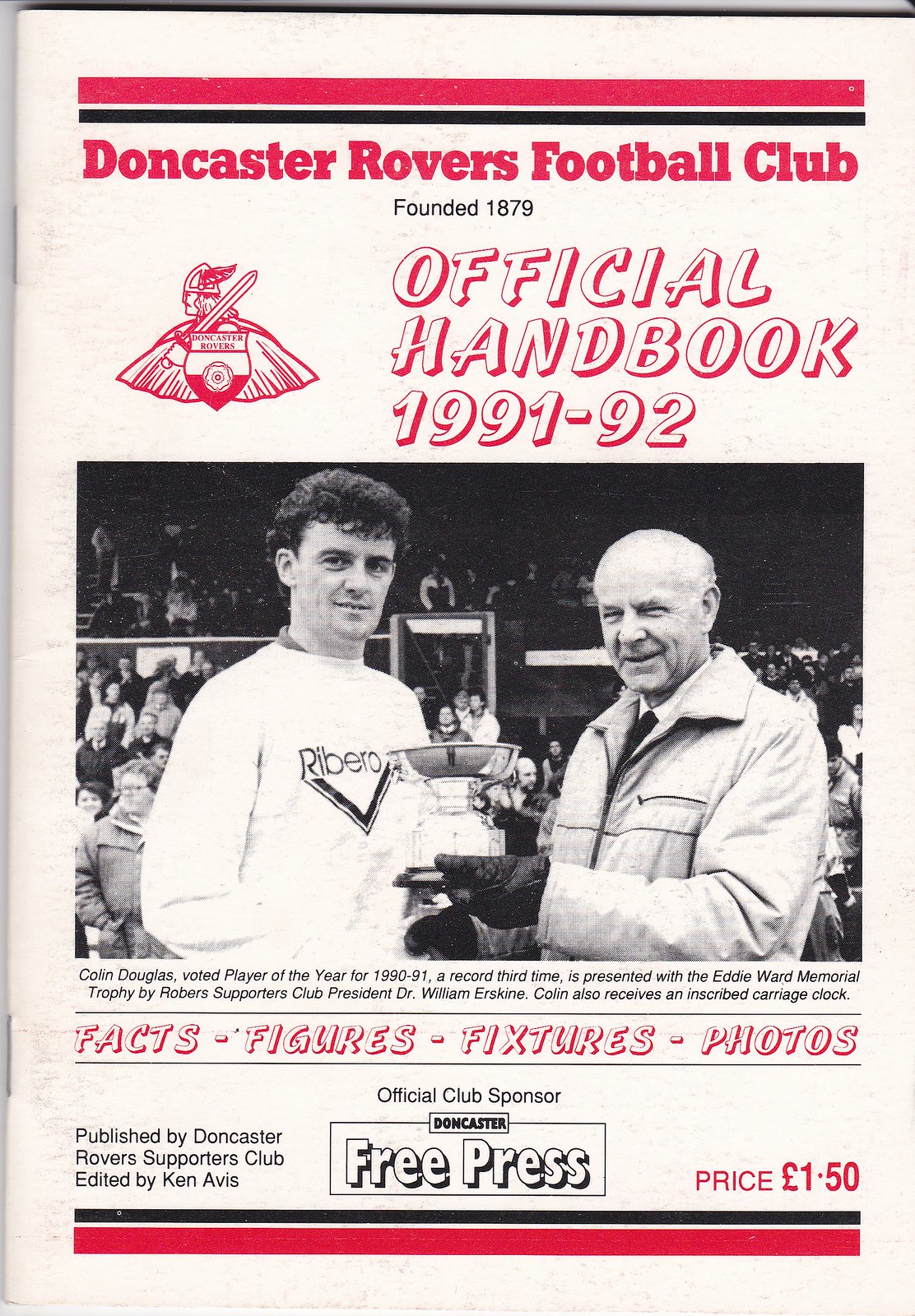The front cover of the official 1991-92 Doncaster Rovers Football Club handbook, published by the Doncaster Rovers Supporters Club and edited by Ken Avis, features distinctive design elements and informative text on an off-white background. At the top, red and black horizontal stripes accentuate the title written in bold red print: "Doncaster Rovers Football Club," accompanied by the founding year, 1879, in black. Adjacent to the club’s winged helmet logo, the subtitle "Official Handbook 1991-92" is inscribed in white text with red outlines.

Dominating the central section is a large black-and-white photograph capturing a significant moment: Colin Douglas, wearing a white sweatshirt with the word "Ribeiro," is receiving the Eddie Ward Memorial Trophy from an older, balding man in a coat and black gloves, identified as the Rovers Supporters Club President, Dr. William Erskine. This ceremony honors Douglas for being voted Player of the Year for 1990-91, marking his record third win. He also received an inscribed carriage clock.

Below the image, in black text, the caption repeats this achievement and presents additional categories "Facts, Figures, Fixtures, Photos" in white text outlined in red. Along the bottom of the cover, further details are provided: it states the publication was edited by Ken Avis, sponsored by the Doncaster Free Press, and is available for £1.50. The layout is framed by additional red and black bars at both the top and bottom, adding to the booklet’s classic aesthetic.